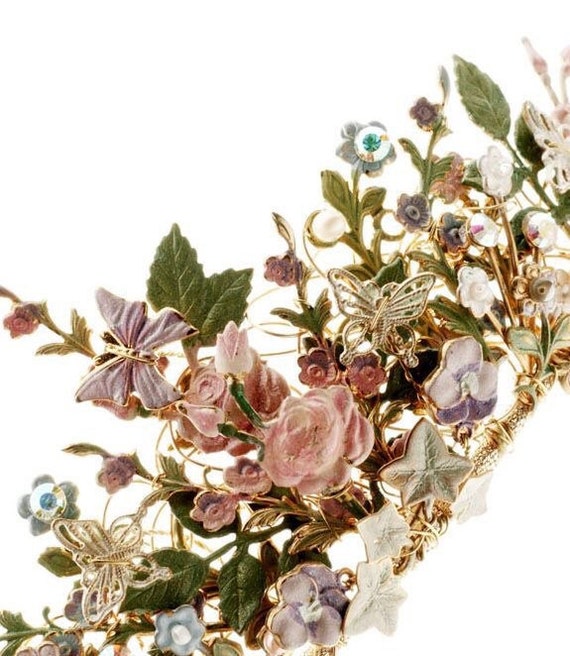The image depicts an intricately designed piece of artwork featuring a diagonal arrangement of metal flowers and butterflies extending from the lower left to the upper right against a stark white background. The composition appears to be a blend of jewelry-like elements, with a decorative gold band or rod serving as a base. From this base, a realistic yet ornamental collection of flowers and foliage emerges, showcasing pink, purple, and blue blossoms, some adorned with tiny jewels. The petals and leaves are outlined in thin gold borders, lending a sense of elegance and richness to the image. Scattered among the flowers are butterflies in shades of pink, purple, and gold, adding vibrancy and movement. The whole arrangement combines elements of metalwork and artistic flair, capturing the look of a sophisticated, metallic display.